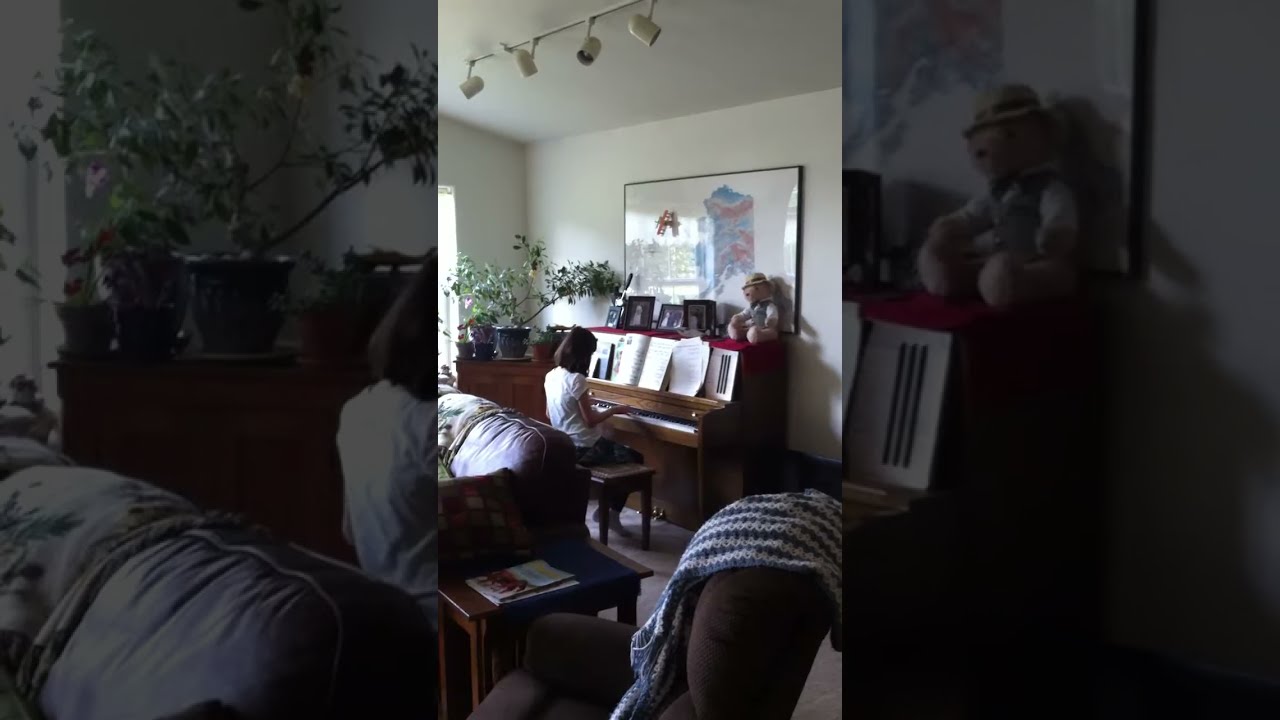In this detailed image, a female dressed in a white shirt and dark pants is playing a light brown piano positioned centrally in her living room. Music books and a small teddy bear are propped up on top of the piano. Behind the piano on the white wall, there's an art piece with a predominantly white background, accompanied by several smaller framed photographs. Over to her left, a window allows natural light to filter in, while a corner cabinet hosts an array of green plants in pots. Above her, four lights are mounted on track lighting.

In the backdrop, a brown couch is partially visible with a small side table beside it. In the foreground, a brown recliner adorned with a striped blue and white afghan faces towards the scene. The room's colors predominantly include shades of brown, white, green, and blue, suggesting a warm and inviting interior. This image encapsulates a cozy indoor setting, with the woman engrossed in her musical pursuit.